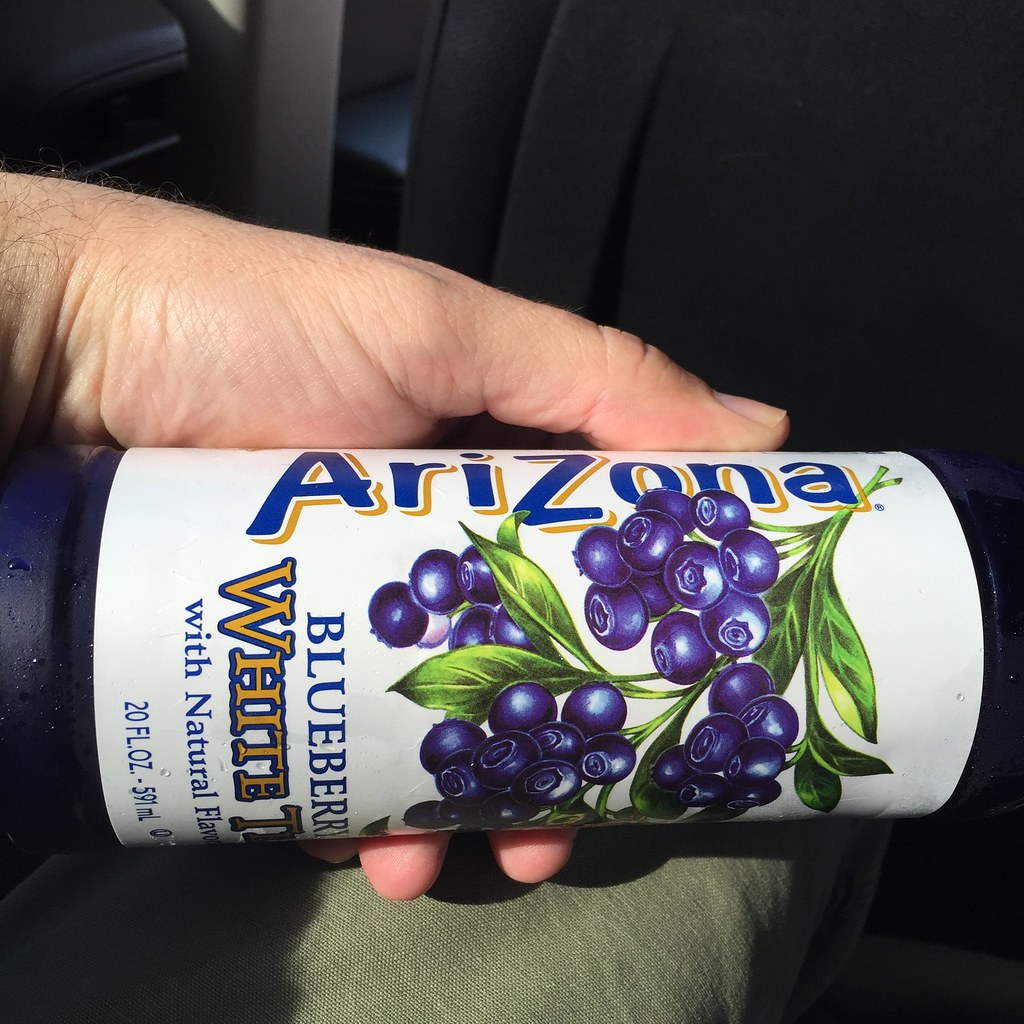In this image, a hand is seen holding a sideways Arizona tea container. The hand enters the frame from the top left corner, with the thumb positioned on top of the can and three fingers wrapped around its underside. The can features a white label with black bands at the top and bottom. From this perspective, the top of the can displays the word "Arizona" in blue text outlined in brown. Below the brand name, there is an illustration of blueberries attached to leafy stems. Further down, the can's label includes the word "blueberry" in blue text, a large "T" in brown, the phrase "with natural flavoring," and "20FLOZ." The backdrop includes a gray pant leg and a black background, adding contrast to the foreground elements.